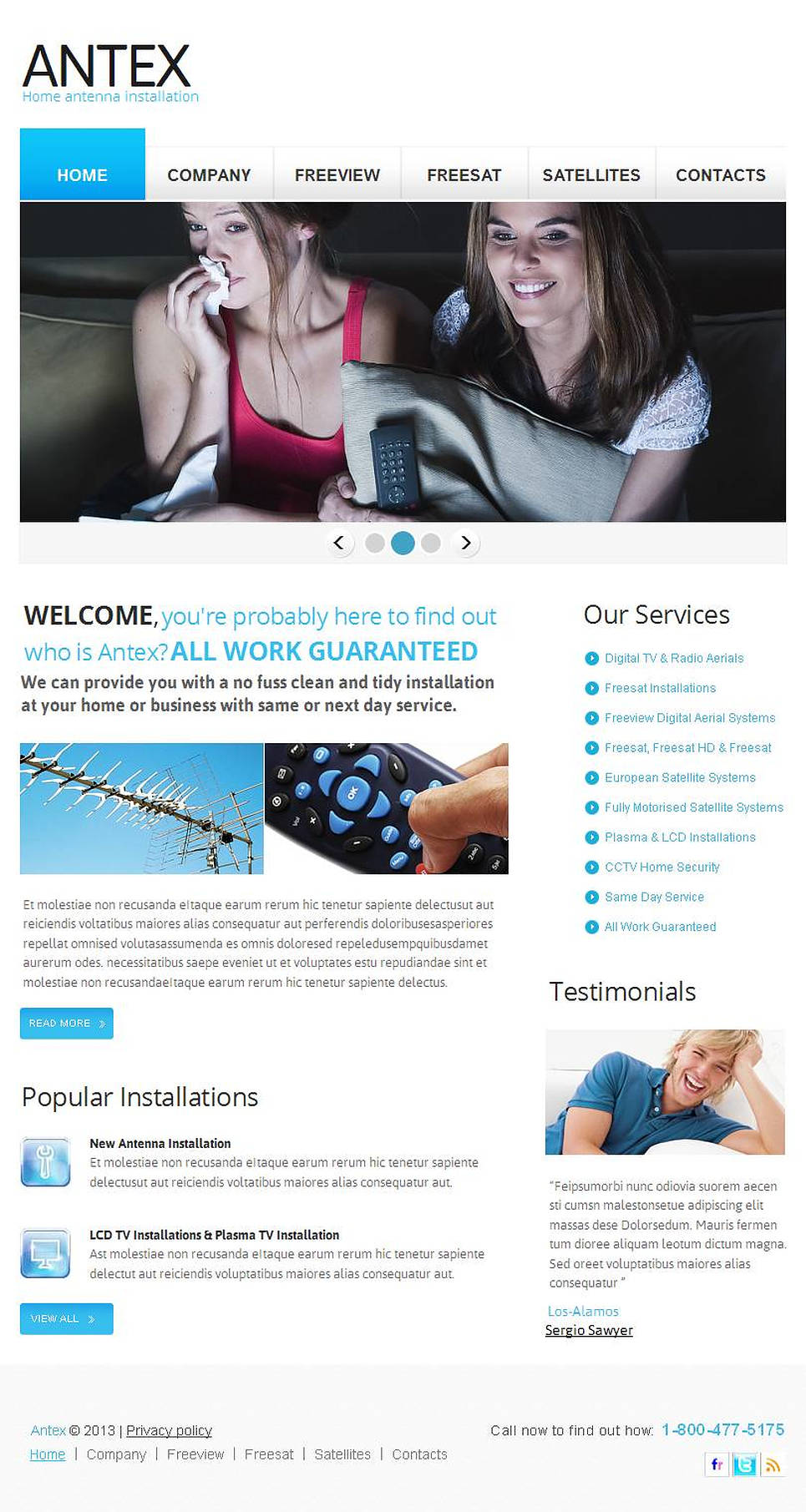The webpage prominently displays "ANTEX" in large, bold, black font at the top, with the tagline "Home Antenna Installation" written below in blue. Across the top of the page are navigation tabs labeled "Home," "Company," "Free View," "Free SAT," "Satellites," and "Contacts." The "Home" tab is highlighted in blue with white text, while the remaining tabs are white with black text.

The central image on the page features two women on a couch watching TV. The woman on the left is wearing a red tank top and is crying into a tissue, while the woman on the right is smiling and hugging a pillow.

Below the image, there is a welcome message that reads: "Welcome, you're probably here to find out who is ANTEX. All work guaranteed. We can provide you with a no-fuss, clean, and tidy installation at your home or business with same day or next day service." 

Following this, there seems to be placeholder text in another language, likely intended for future content. Further down, there are highlighted service offerings: "Popular Installations," including "New Antenna Installation," "LCD TV Installations," and "Plasma TV Installations." Once again, there is placeholder text, suggesting areas meant for additional details or descriptions.